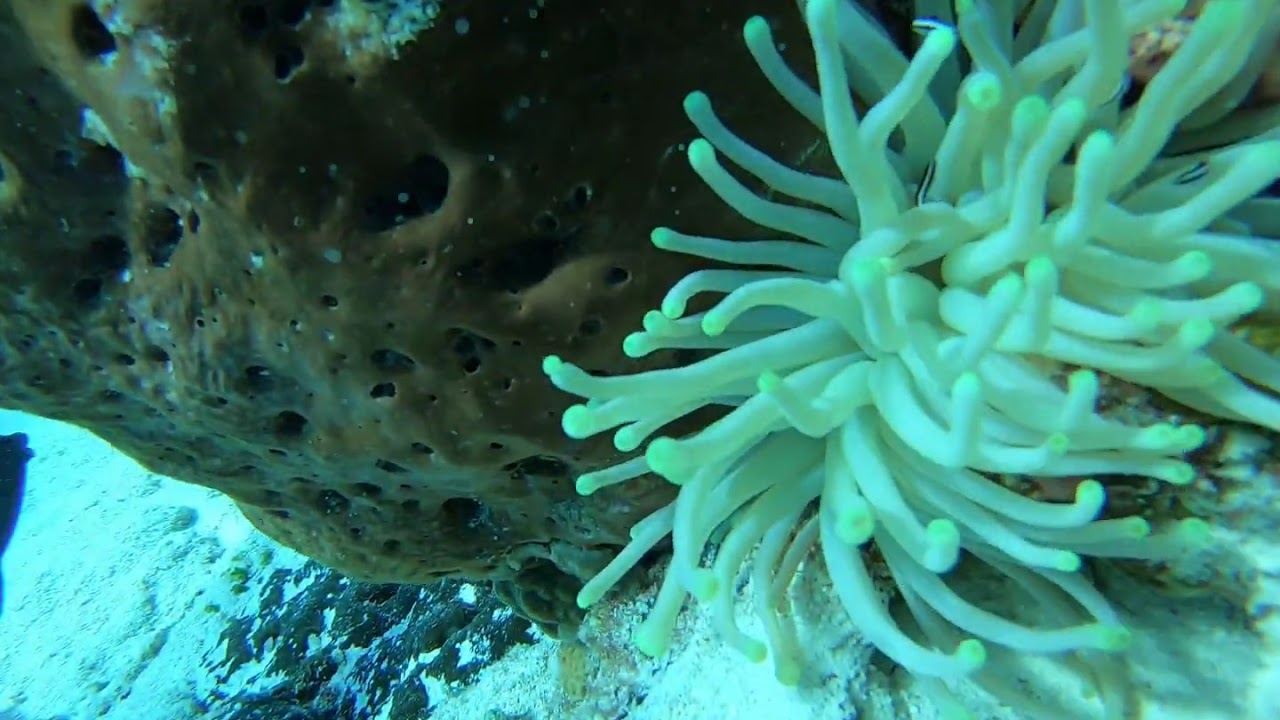The image depicts an underwater scene likely taken through the window of an aquarium, given the distinctive lighting and clarity. Dominating the left side, there is a large, dark brown piece of coral or a rock with holes, resembling coral structure. On the right side, a bright, almost neon, teal-colored sea anemone with thin, tubular, spaghetti-like tendrils captures attention. The ocean floor below consists of fine white sand scattered with some larger black rocks. Further to the left, part of a fish’s head is visible, peeking into the frame. The lighting casts a light bluish-teal hue over the entire scene, enhancing the aquatic ambiance.